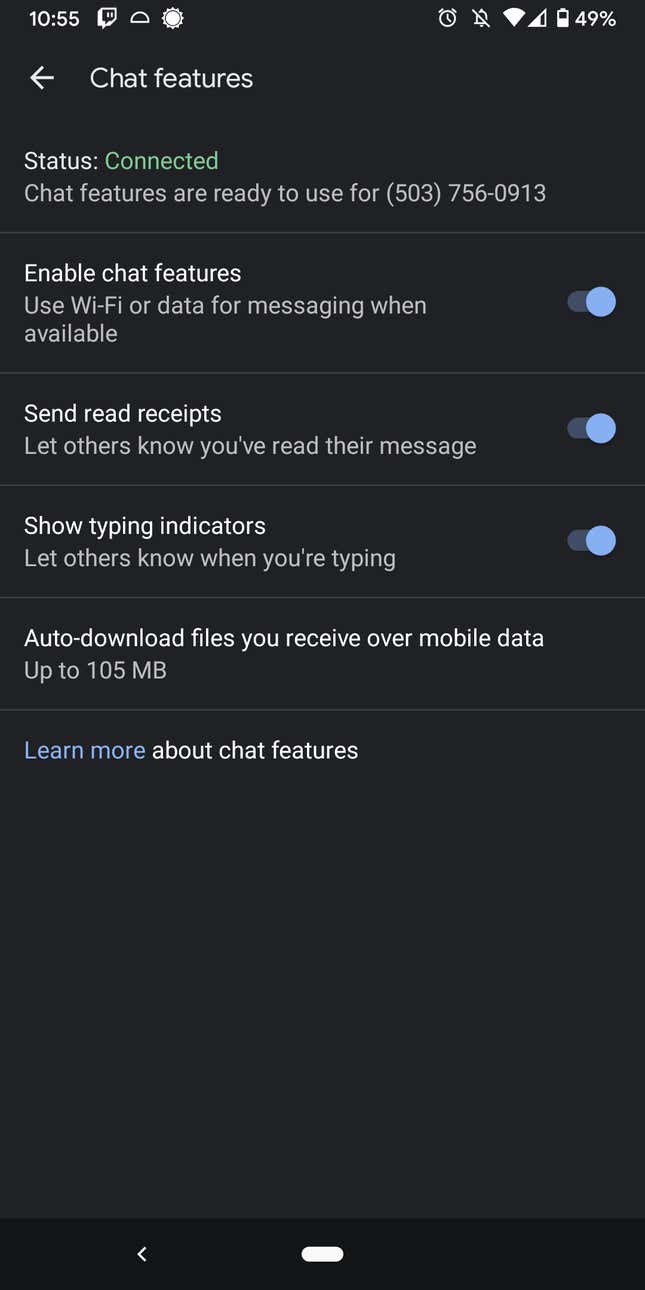The image is a dark gray rectangular screen resembling a smartphone interface. In the top left corner, the time "10:55" is displayed, accompanied by a half-circle symbol and a sun-like icon. On the right-hand side, there is an alarm clock, a bell icon with a line through it, a WiFi symbol, and a triangle pointing left that broadens towards the right. 

A battery icon, half-filled, shows a charge of 49%. Below this, an arrow pointing left is next to the text "Chat Features." The status line reads "Status: connected," with "connected" highlighted in green. Further text informs in white: "Chat features are ready to use for (503) 756-0913," followed by a gray separator line. 

Moving down, it prompts to "Enable chat features: Use WiFi or data for messaging when available." Below this, a dark green bar with a light green circle next to it reads "Send read receipts: Let others know you are reading their messages." 

Another section features a dark blue bar and a larger light blue circle with the label "Show typing indicators: Let others know when you are typing." There is an option to "Auto-download files you receive over mobile data up to 105 MB," followed by a white separator line. 

At the bottom, a blue link says "Learn more about chat features." Finally, a blank space precedes a black rectangle containing an arrow pointing left and a white bar.